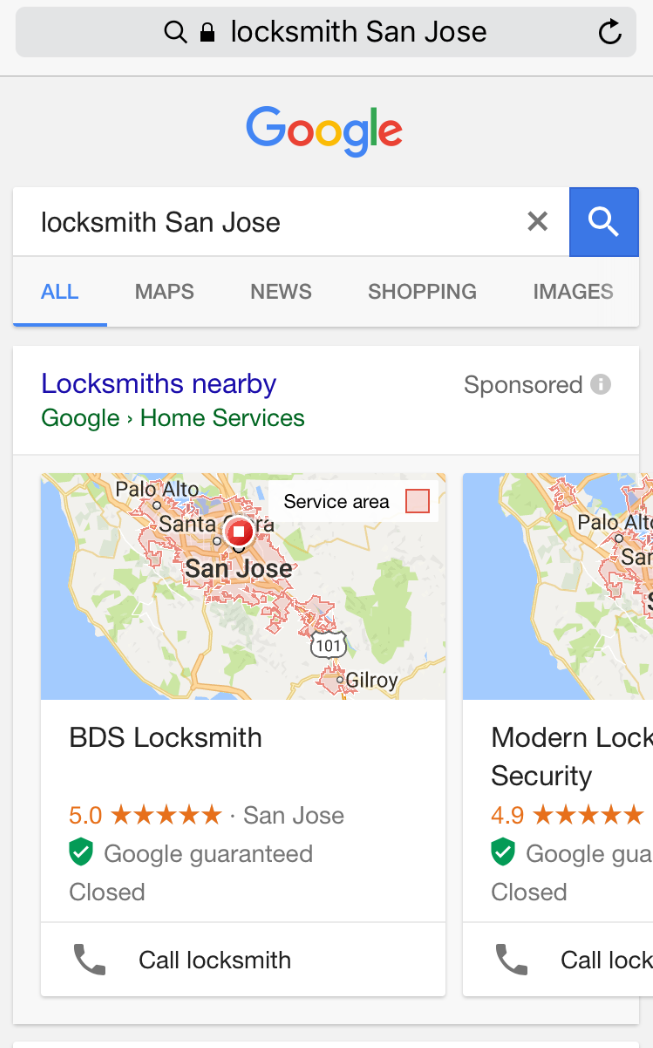Screenshot of a Google search page for "locksmith San Jose." At the top, there is a search field containing an icon for search, a lock icon, and the text "locksmith San Jose." To the right, there are refresh and settings icons. Below the search field, there's a gray line followed by the Google logo in its signature blue, red, yellow, and green colors. Below the logo, there's another search bar displaying "locksmith San Jose" with a clear ("X") button on the right and a blue search button with a white magnifying glass icon.

Underneath the second search bar, various tabs are available: All, Maps, News, Shopping, and Images. The "All" tab is highlighted in blue with a blue underline, indicating it's the active tab, while the rest are in gray. Below the tabs, the search results show "Nearby locksmiths" and "Google Home Services." "Nearby locksmiths" is highlighted in blue, and to its right, "Sponsored" is displayed with an information icon (an "i" in a circle).

A map of San Jose is shown below the tabs, with markers indicating the locations of locksmiths. The visible results include a listing for "BDS Locksmith" with a 5-star rating in San Jose, California, marked as Google Guaranteed and showing that it is currently closed, with an option to call the locksmith. Right below, there's another listing for "Modern Locksmith Security" with a 4.9-star rating. Only one and a half listings are fully visible, suggesting there are more listings accessible by scrolling or swiping.